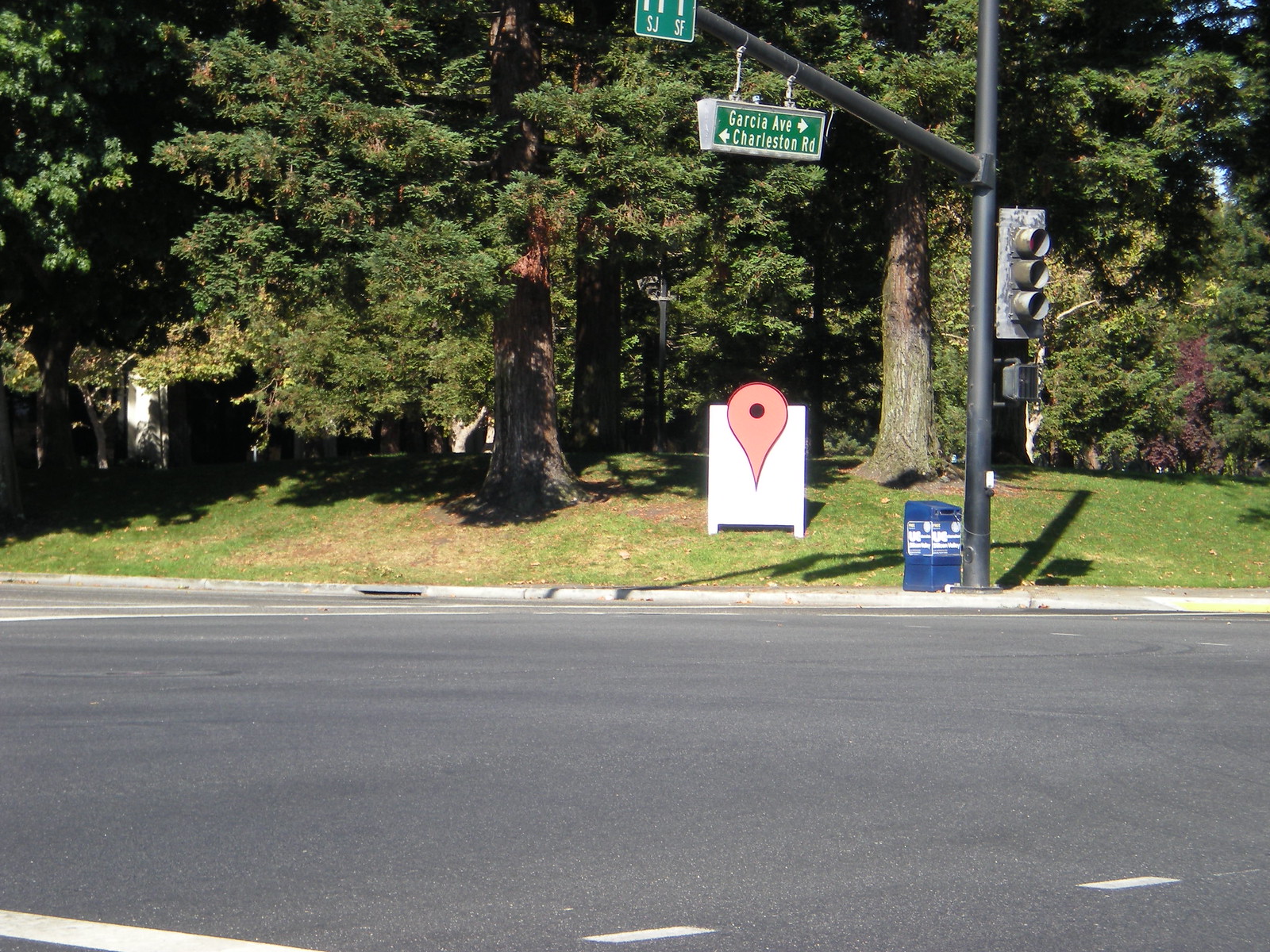A picturesque scene captured outside with a backdrop of lush, green pine trees standing tall with their dense foliage and brown trunks, indicative of the summer season. The trees do not show any signs of brown leaves, emphasizing the vibrant greenery. In the foreground, a gray paved road runs horizontally, devoid of any vehicles. The road features white lane markings separating two lanes. Between the lush trees and the road lies a strip of well-kept green grass, which is bordered by a pristine white curb. Adjacent to the curb, there is a street sign and a traffic light mounted on a dark gray pole. From this pole, a green street sign hangs, suspended by short chains. The sign bears the names "Garcia Avenue" with an arrow pointing to the right and "Charleston Road" with an arrow pointing to the left, all in white text. Below the street sign and next to the pole, there is a blue box with white text, possibly a mailbox or a trash can, completing the well-maintained suburban scene.